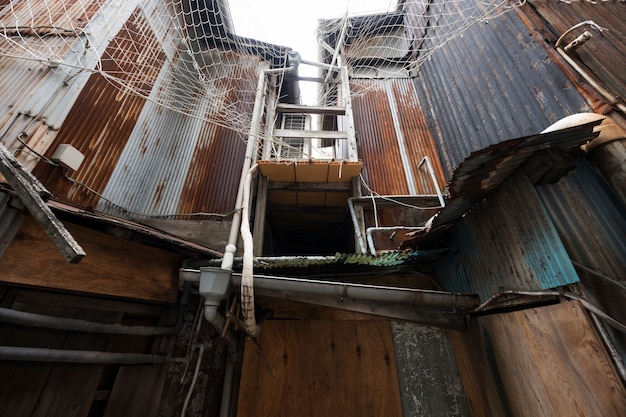In this ground-level photograph, we look upward at a dilapidated structure predominantly made of rusted metal and aged wood. The metallic elements, which may be purlings or thin metal plates, exhibit significant rust and are interspersed with patches of white and black. These metallic components form the makeshift walls and roofing of what appears to be a shanty or slum-like dwelling. Scattered among the metal pieces are brown and dark brown wooden elements, likely part of a deteriorated stairway. Above the structure, a netting, possibly resembling a fishing net, is visible, hanging loosely in the whitewashed sky. The image also features pipes protruding from the buildings and rain gutters that are nearly torn off, further emphasizing the decay and neglect of the place. The dark voids behind the structural openings indicate the inner recesses of these homes or apartments. The photograph, devoid of any text, captures a scene of rust, wood, and looming degradation.